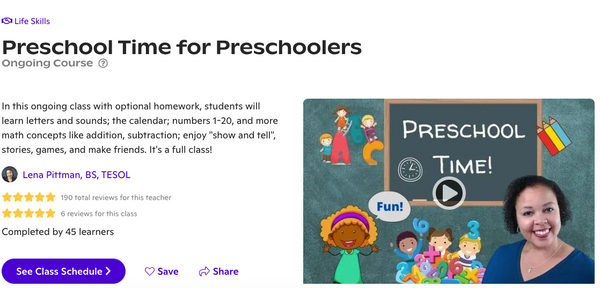In the top left corner, the background is a vibrant purple color announcing the "Pre-School Time for Pre-Schoolers" class. This ongoing class, which includes optional homework, is designed for young children to learn letters and sounds, count letters and numbers from 1 to 20, and grasp basic math concepts like addition and subtraction. The students will also engage in activities such as show and tell, storytelling, games, and making friends. It's evident that this is a popular and full class.

The teacher for this class is Lena Pittman, who holds a B.S. in TESOL. She has been highly rated, with 112 reviews for her teaching and an additional 6 reviews specifically for this class, completed by 45 learners. The teacher’s credentials are highlighted by five gold stars.

The purple section also indicates where to see the class schedule. The description includes various interactive elements and colored visuals. There’s an image detail with a person in a blue shirt and red pants, another figure portrayed in purple standing up, and something orange in the scene.

The backdrop of the image resembles a chalkboard, adding an academic feel, and is decorated with colored pencils in red, yellow, and blue. Another focal point is a teacher standing on the right side of the image; she has short curly hair, is smiling warmly, and wears a blue shirt with necklaces. The scene conveys a fun and engaging learning environment, emphasized by numbers and playful elements scattered around.

Overall, the detailed description illustrates a vibrant and interactive pre-school class led by a well-reviewed and enthusiastic teacher.